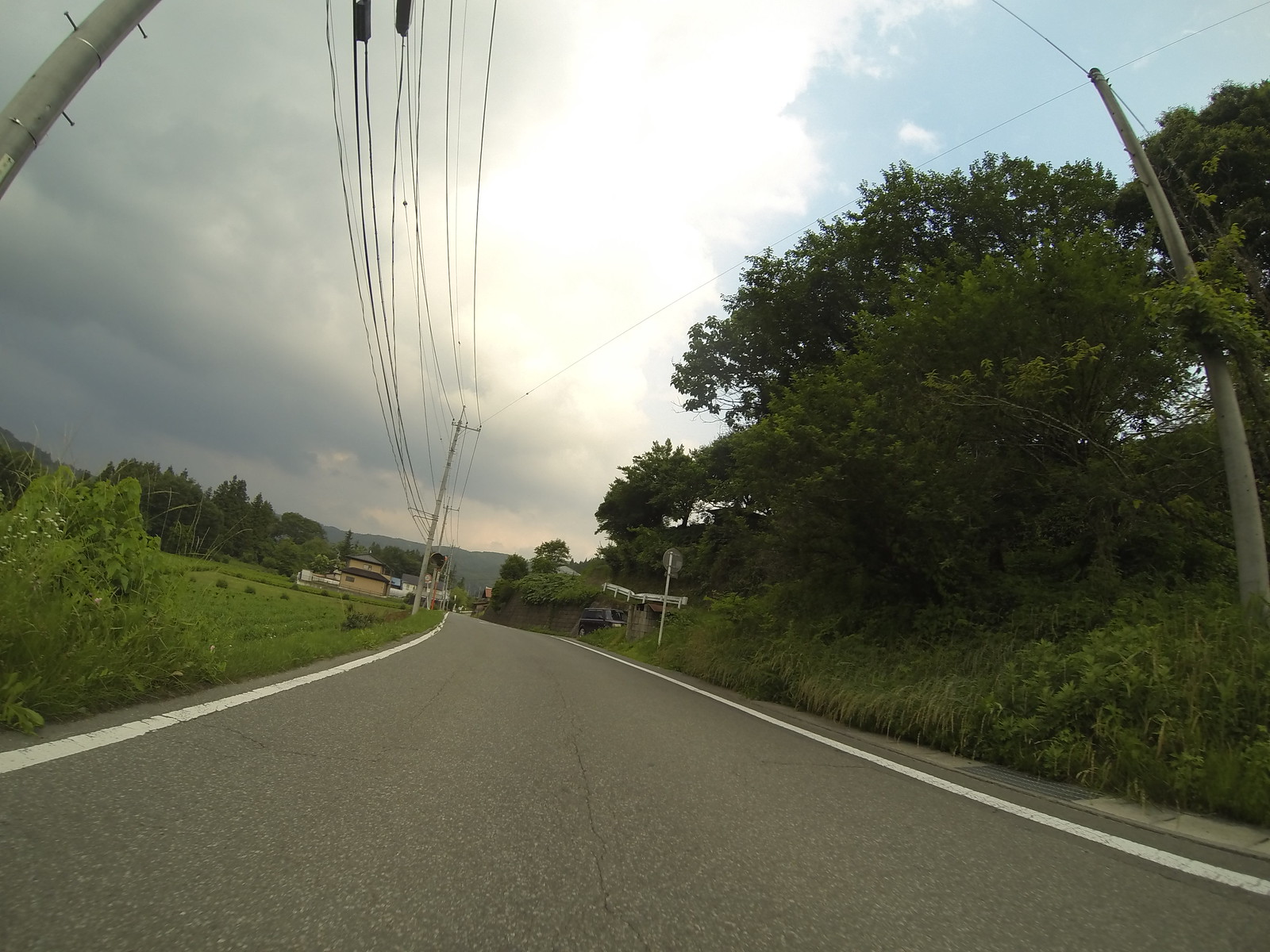This photo, taken from approximately knee level with a fisheye lens, depicts a paved country road stretching into the distance. The light gray pavement features white side lines, and the emptiness of the road underscores its serene, rural setting. On the right side, a grassy hill dotted with trees slopes upward, while the left side reveals a flat grassy field. Telephone and power lines are visible along the road, which contribute to the sense of infrastructure in this otherwise sparse scene. In the distance, beige and white houses with brown roofs are visible, alongside a stop sign and a parked car by a brown retaining wall. An additional vehicle is parked at a turnout area further down the road, adding a touch of life to this quiet setting.